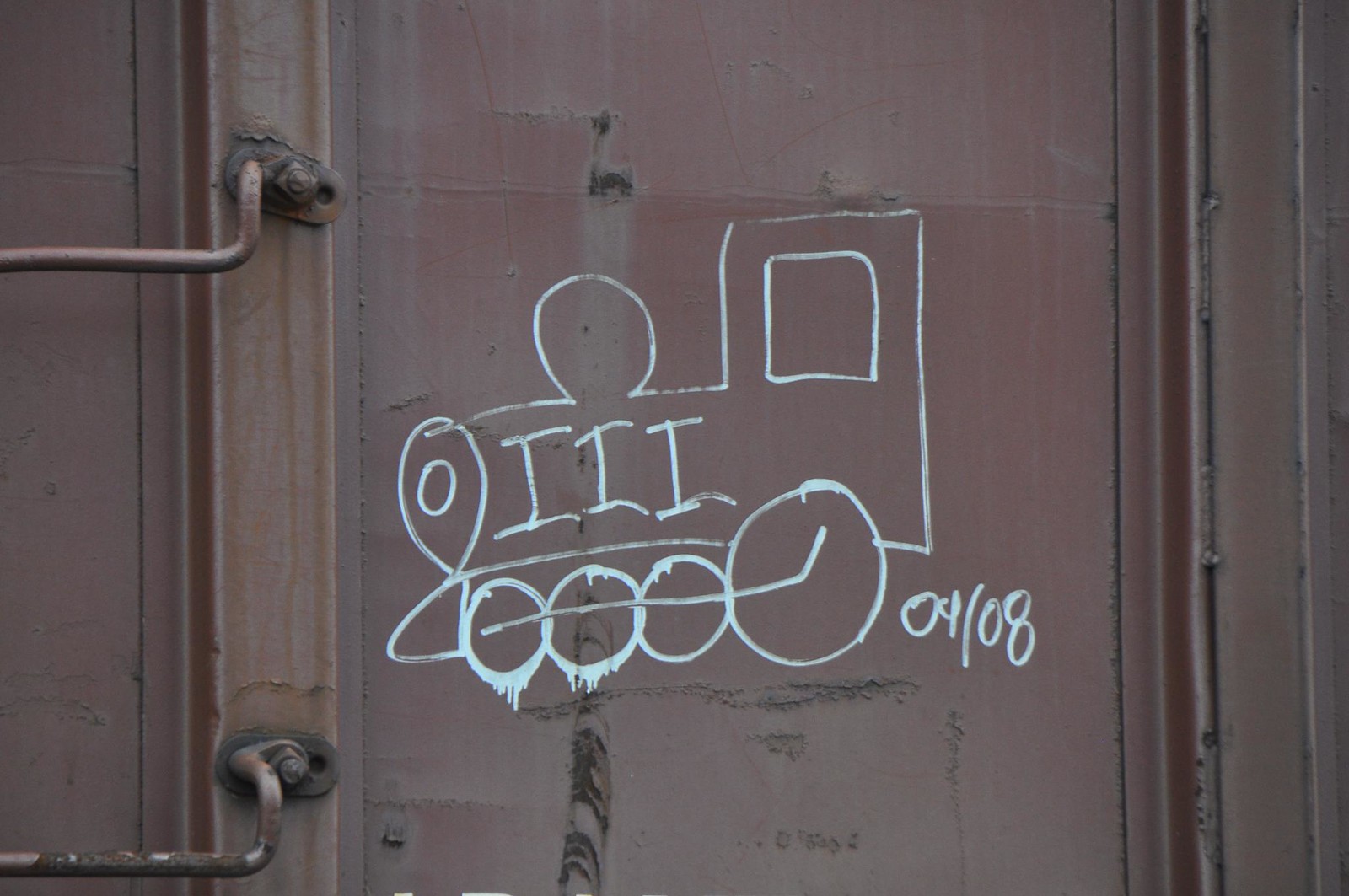This photograph captures a rusted, industrial brown door, possibly from an establishment or a train car, adorned with intricate graffiti. The centerpiece of the graffiti is a childlike drawing of a train, sketched in a dripping white or tainted sky-blue marker. The train features four interconnected wheels and a distinctive front marked by a giant hole. Above the wheels, the body of the train showcases three capital 'I's that resemble three eyes. On the bottom right corner of the train drawing, there is a date inscribed as "04/08" or "09/08," further adding to the character of the artwork. The surrounding area of the door is marred by rust and giant bolts, enhancing the gritty, industrial aesthetic of the scene.